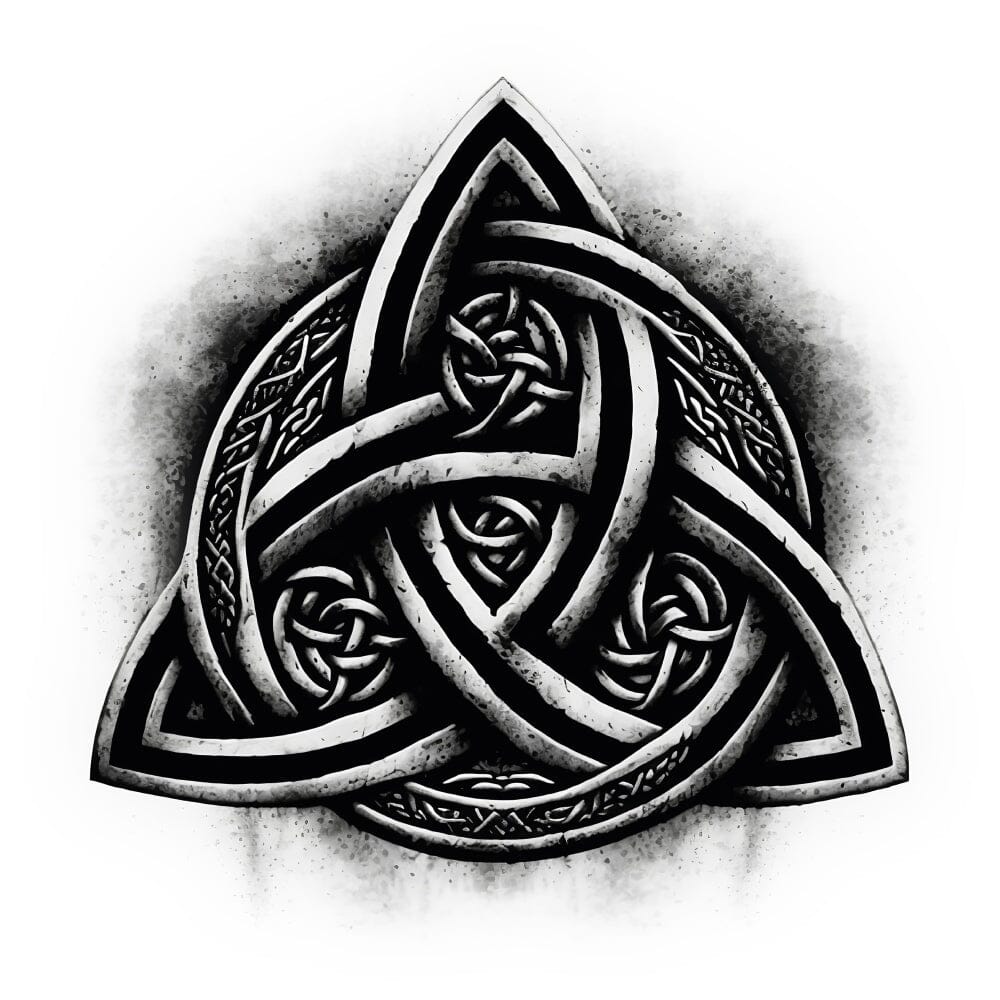The image features a detailed black and silver gray Celtic trinity knot, known as a triquetra, set within a hazy black background. The design centers around a circle bordered by gray on both its inner and outer edges, containing rows of intricate, intertwined vines. Enclosed within the circle, three seamlessly connected pointed loops create a continuous, flowing pattern. One loop extends from the very top, arcs downward behind the circle to the lower right, then curves back through the center toward the lower left, creating a pointed tip before looping back behind the circle and completing the top point. Each loop has silver or gray borders with black inner sections, forming a harmonious interplay of colors and shapes. In between these loops, small twisted knots occupy the open spaces, adding to the complexity of the design. The background fades outward from a dense black spatial corona, enhancing the visual depth and focusing attention on the central triquetra. This emblematic design gives off a metallic, steel-like appearance, further accentuating its intricate craftsmanship.